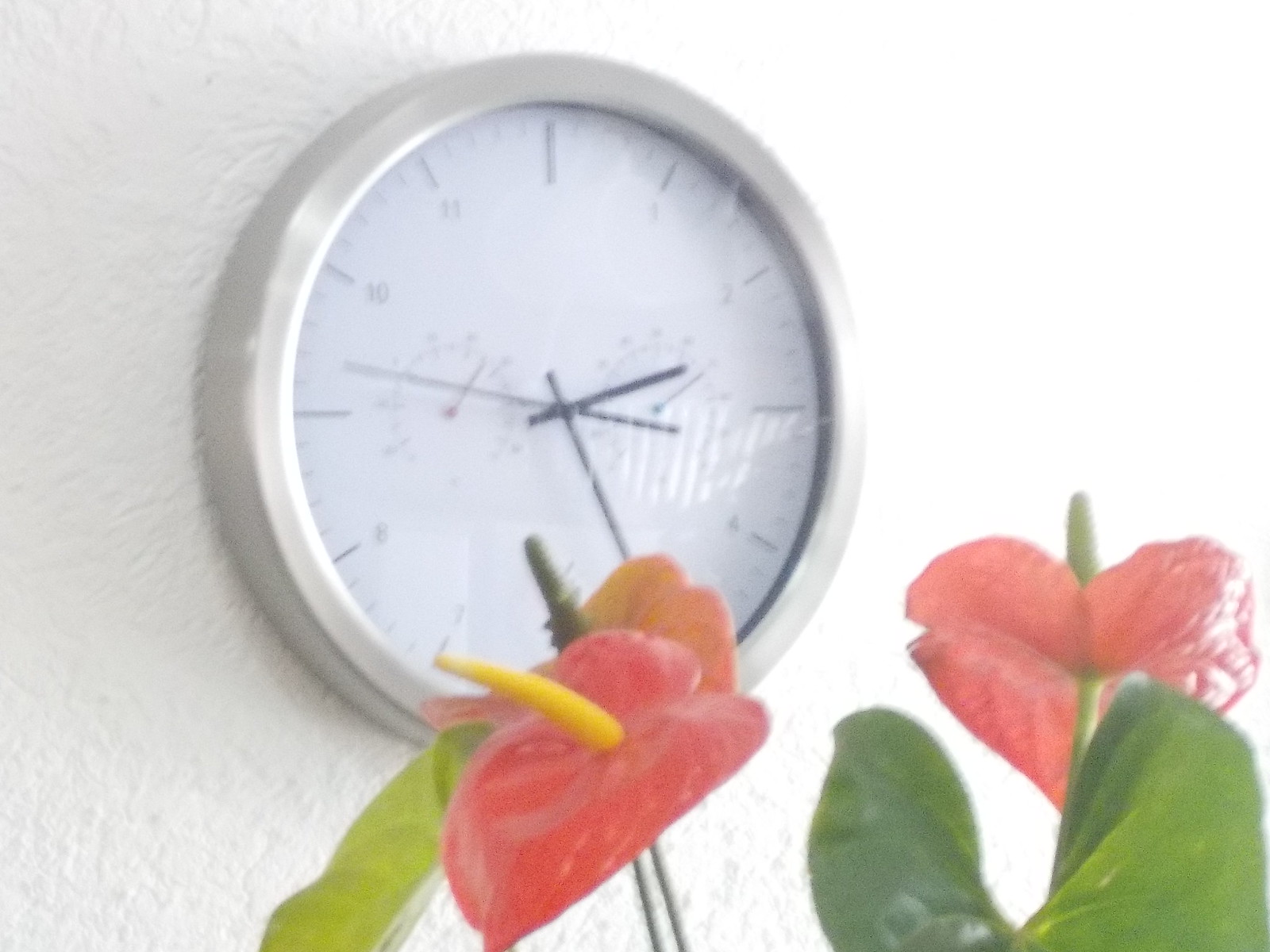A circular wall clock with thick silver edges is mounted on a pristine white wall. The clock's face is a stark white, featuring two smaller dials reminiscent of a classic chronometer, presumably for measuring minutes and seconds. Beneath the clock, a cluster of artificial plants adds a touch of nature. The plants boast green leaves and pinkish blooms, each adorned with yellow and green horn-like structures protruding from their centers.